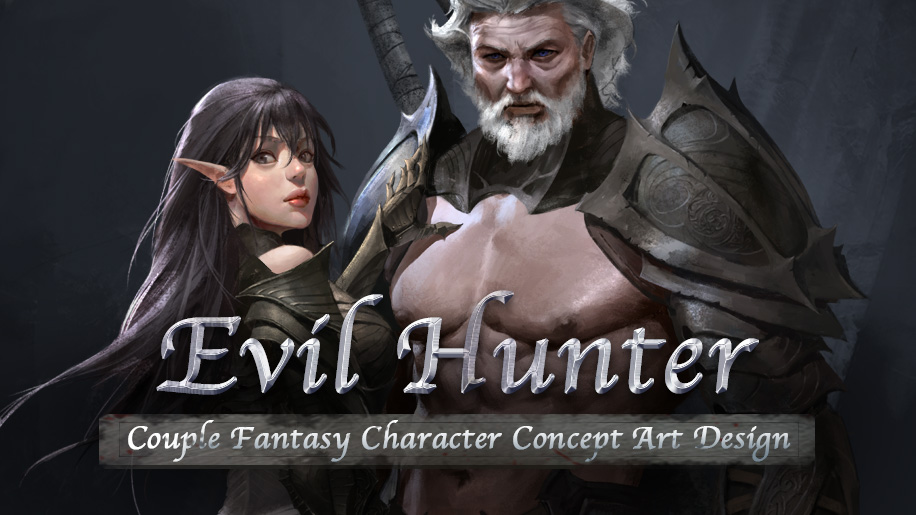The image is a horizontal, digitally drawn artwork that resembles a poster, potentially for a video game or anime series. Centered are two characters, a muscular older man with a fierce gaze and a woman with an elegant demeanor. The man, with white hair and facial hair, is looking straight ahead. His intense blue eyes are unmistakable, and he has a bare chest with brown armor on his arms and shoulders. He also appears to have a long weapon strapped behind his back. 

Beside him, the woman has long, straight black hair with bangs that frame her face, pointed elf-like ears, and wears subtle lipstick. She's dressed in a greenish uniform and is looking directly at the viewer, her body turned slightly to the right. 

Dominating the center of the image, in bold white letters, is the title "Evil Hunter." Below this, in smaller print within a gray rectangular box, the text reads "Couple Fantasy Character Concept Art Design." The backdrop is a dark gray, nondescript wall that enhances the prominence of the characters.